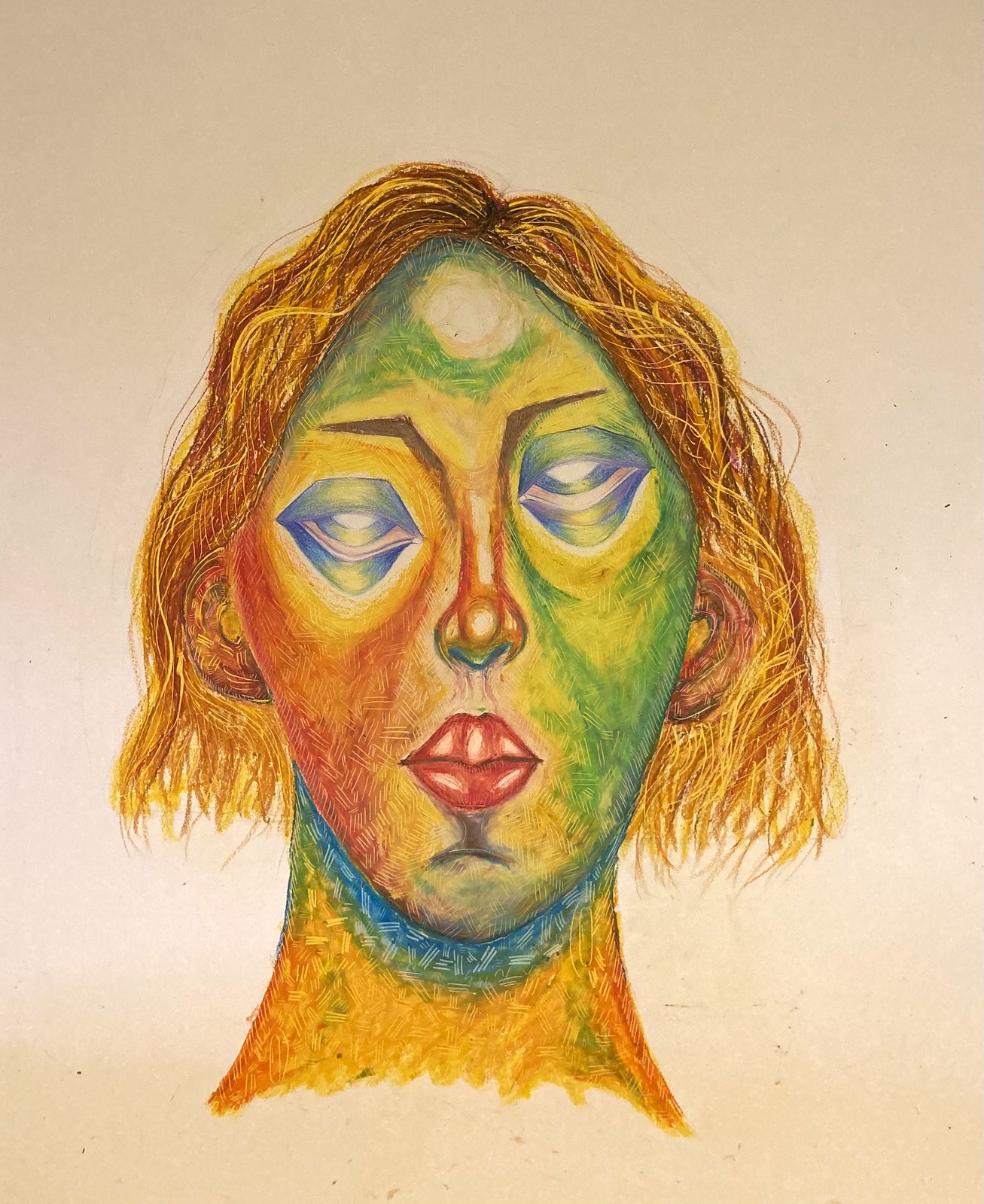This image is a striking, abstract portrait of a woman with an oval-shaped face, viewed directly forward. Her face is divided into two vivid colors: green on the right and yellow-orange on the left, with a subtle red shading on the right side. The eyes are intentionally asymmetrical, with the left eye lower than the right, each featuring white sclera and blue-green eyelids. She has tall, red lips that sit above a red area suggesting either a pedestal or a goatee-like design. Her nose is long and thin, and her eyebrows are angular, crafted with a sharp black line. Her hair, parting down the center, appears shaggy and stringy, blending shades of blonde, yellow, and brown, while a white circle highlights the top of her head. A distinct shadow underneath her face transitions from dark blue to yellow at the neck, which also shows a blue handkerchief-like element. The background of the portrait is a raw gray or beige paper, accented with darker speckles, giving the image a textured depth. Overall, this artistic piece combines human and alien-like features, showcased with vibrant, contrasting colors and geometric shapes.